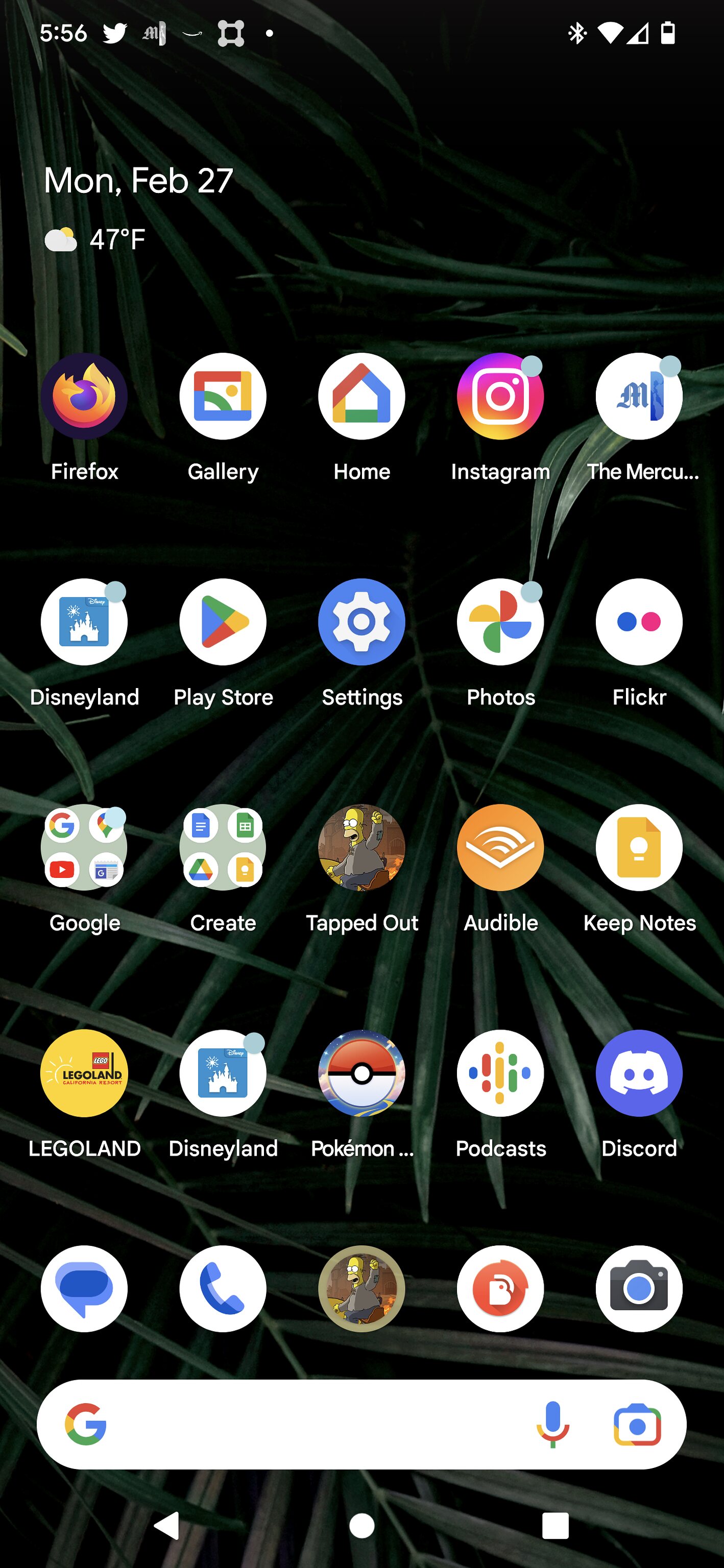The image displays a digital screen with a black background, structured in a triangular layout. At the top left corner, the date "Monday, March 27th" is prominently displayed in white font. Directly beneath the date, an icon of a cloud is shown, accompanied by the temperature reading "47°F". Below this information, there is an orderly arrangement of app and program logos, organized into five distinct rows. At the bottom of the screen lies the Google search bar. 

In the first column from the left, the logos are as follows (top to bottom): Disneyland, Play Store, Settings, Photos, and Flickr. The second column includes icons for Google, Create, Tapped Out, Audible, and Keep Notes. The third column features icons for Legoland, Disneyland, Pokémon, Podcast, and Discord. In the fourth column, subsequent to the app logos, there is a search icon, a phone icon, a circular photo, and another icon characterized by a red circle with a white "B" in the center, followed by a camera icon depicted as a white logo with a black camera in the middle.

Directly under the Google search bar at the bottom of the screen are three navigation icons: a white arrow pointing to the left, a white circle in the middle, and a square white box on the right.